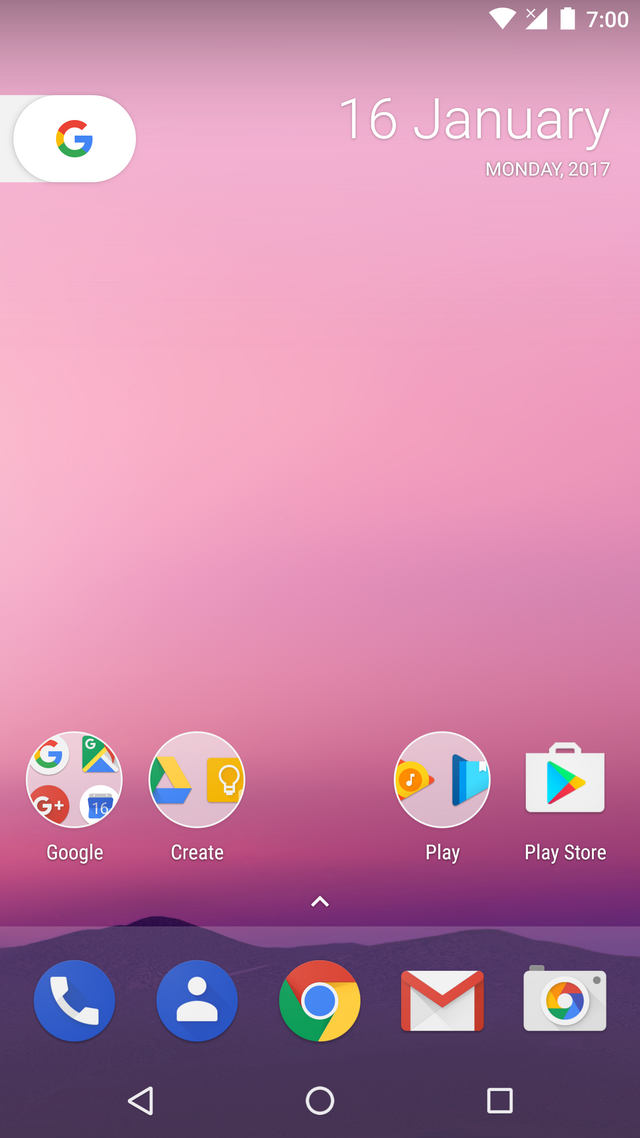The visually compelling image starts with a captivating gradient background. At the top, a light pink hue immediately draws attention, which then seamlessly transitions into a darker pink-purple blend. Near the bottom, the gradient reveals what resembles undulating purple hills, with a few dark purple peaks extending above a horizontal line, creating the illusion of distant mountain tops.

In the upper right corner, the image shows a timestamp reading 7:00 and a vertical white battery icon. Below this, the date is listed: "16th, January, Monday, 2017."

On the left side, the Google "G" icon is prominently positioned. Beneath it, starting from the left, a circle encapsulates the word "Google." Adjacent to this, another circle contains a yellow square with a light bulb inside, labeled "Create." Next to this, a circle with an orange music note above the word "Play" is visible. Finally, a white briefcase icon featuring the Google arrow is labeled "Play Store."

Towards the bottom, you'll find a series of blue circles, each representing a different function: a phone, a person's silhouette in white, and the Google Chrome icon featuring red, yellow, blue, and green colors. Lastly, there's the Google Mail icon, followed by a camera icon with a central circular element composed of yellow, red, blue, and green colors.